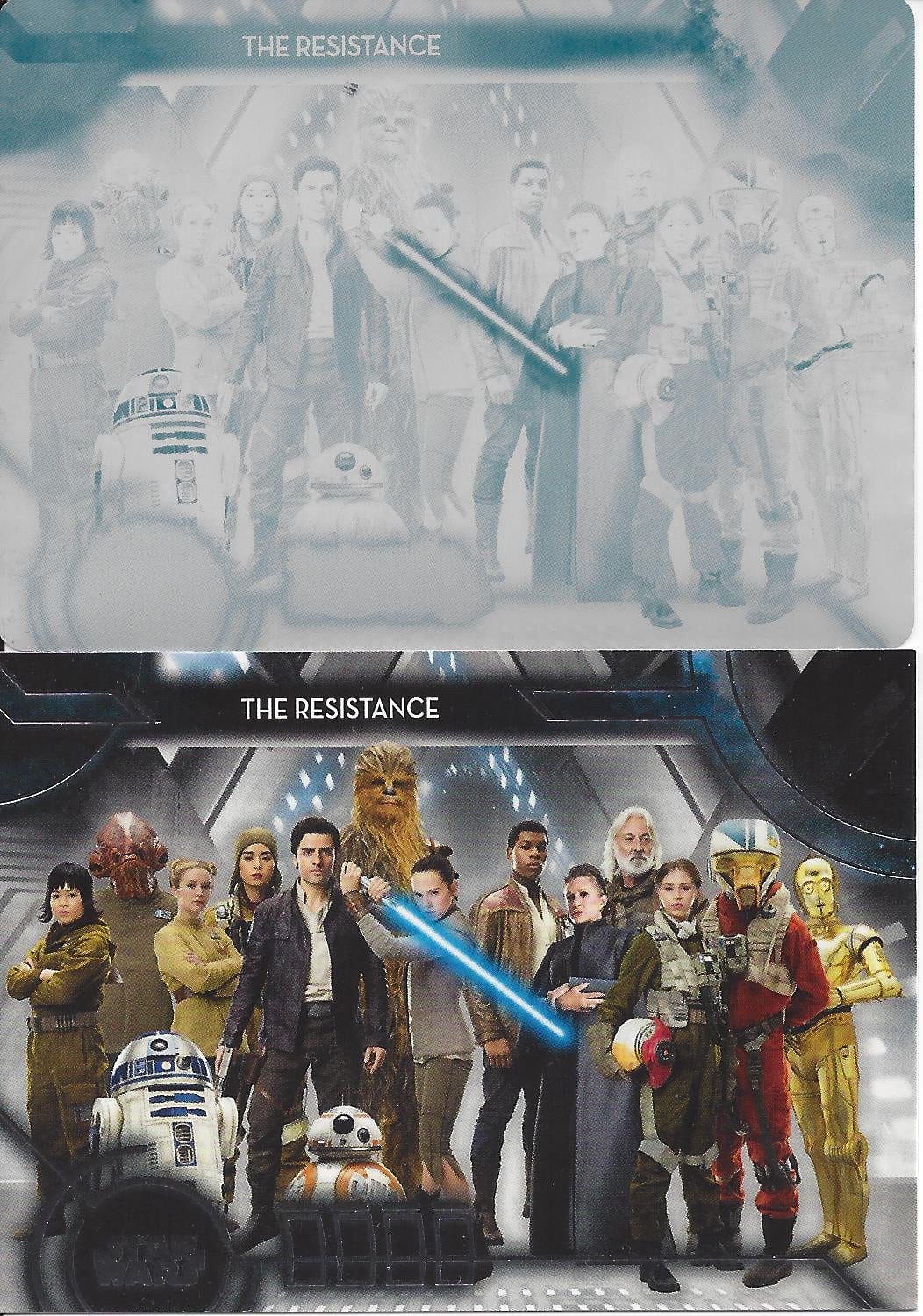The image is a long, horizontally split composition featuring characters from the newer Star Wars movies. The lower half is a vividly colored depiction of these characters lined up shoulder to shoulder, set against a metallic background that resembles a spaceship interior. In the front, R2-D2 stands prominently to the left with BB-8 beside him. Moving back through the lineup, you see iconic figures like Chewbacca, Princess Leia, a central figure wielding a blue lightsaber, and C-3PO situated on the far right. Above this scene, a black box features the words "The Resistance" in white text. The upper half of the image mirrors the bottom but is covered with a white and blue filter that obscures the details, creating a foggy, black-and-white appearance.